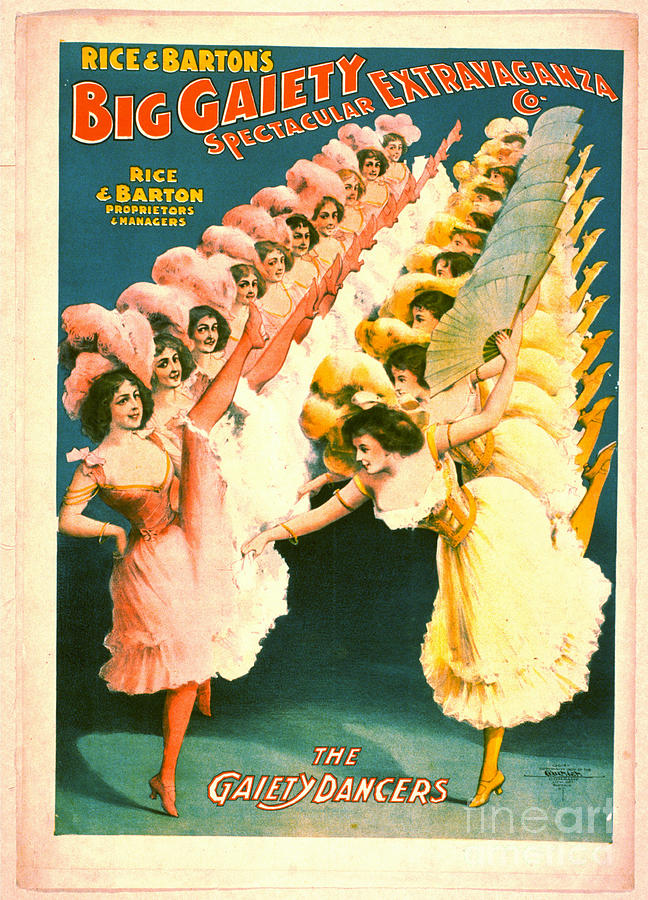This vintage poster, possibly for a theatrical performance, displays muted yet elegant colors. At the top, it prominently features "Rice and Barton's" in yellow, followed by "Big Gaiety Spectacular Extravaganza" in red. Below, it reiterates "Rice and Barton, Proprietors and Managers" in yellow. The central artwork portrays two rows of showgirls in coordinated dance poses.

On the left, a line of dancers in pink frilly knee-length dresses don big hats adorned with pink plumes. These dancers, all sporting pink leggings, heeled shoes, and occasionally seen with a garter, kick high with one leg, creating an energetic display. Conversely, on the right, another row features dancers in corseted yellow dresses, yellow socks, and shoes, each holding a fan in their right hand while kicking back their right leg. The bottom of the poster reads "The Gaiety Dancers" in white. The symmetrical arrangement of dancing figures lends a sense of rhythmic motion, capturing the essence of an early 20th-century spectacular performance aimed at drawing in audiences.